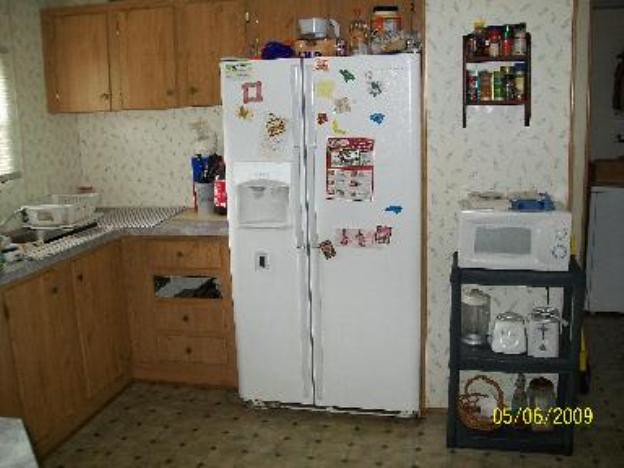This manual photograph, dated 05/06/2009 in yellow text at the bottom right corner, captures a well-used kitchen. In the center of the image stands a white refrigerator, adorned with various colorful magnets and stickers, including green, blue, yellow, and a distinctive pinkish-red square. Clutter is visible on top of the fridge, such as jars, a white Brita filter, and other miscellaneous items. 

To the right of the fridge, a white wall with a grayish marked design hosts a dark wood spice rack filled with an assortment of spices. Below this spice rack, a white microwave rests on a black shelf, accompanied by a blender base, a toaster, and canisters, possibly of flour and sugar. On the left side of the fridge, the kitchen is outfitted with medium wood grain cabinets featuring round circular wood knobs, and a gray countertop with various items like dish mats, a dish caddy, utensils, and a bottle of soda. 

Further left, above the sink, which is silver in color, there's a window providing a natural light source to the kitchen. Overall, the kitchen appears well-lived-in, with signs of daily use and personal touches throughout.